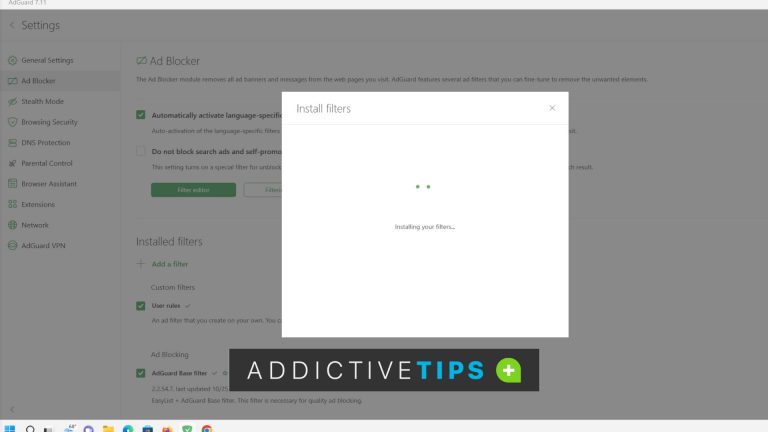This image is a screenshot from a website with a white background, partially obscured by a pop-up in the center. The background has a slight gray overlay due to the pop-up. At the top of the pop-up, there's a gray border with text in the left corner that reads "AdGuard 7.11". 

Below the gray border, on the left side of the pop-up, there is a dark gray section with a shadowy appearance. Here, you can see the word "Settings". Beneath this, there is a vertical list of icons, each corresponding to different tabs. The second icon down is highlighted, indicating it’s the currently selected tab, labeled "Ad Blocker".

To the right of these icons, the content related to the "Ad Blocker" tab is displayed. At the top left of this section, it says "Ad Blocker" followed by a dividing line. Underneath this heading, there's a green square with a white check mark next to the text "Automatically activate language-specific filters". Below this, another square, which is unchecked, reads "Do not block search ads and self-promotion".

Further down, partially obscured by the pop-up, there are buttons including a green one (unreadable text) and a white one. Below these buttons, it says "Installed Filters" followed by details about the installed filters. In the center, there's a white square with "Installed Filters" written in black text in the top left corner and a black 'X' in the right corner. Just below, there's another black section with two dots and the text "Installing your filters...".

Towards the bottom of the pop-up, a black rectangle about three inches wide contains bold text. Inside this rectangle, in white capital letters, it says "ADDICTIVE", followed by bold blue capital letters "TIPS". Next to this text is a green circle with a white plus sign inside.